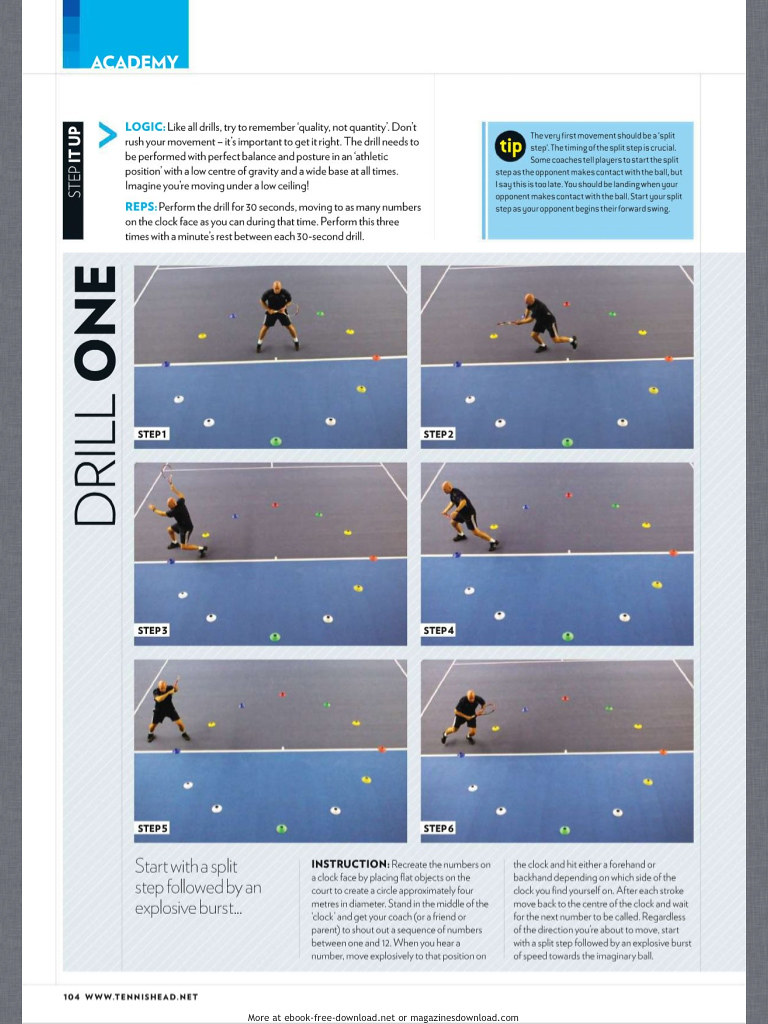This is a detailed color photograph of a page from an instructional book or magazine, likely focused on sports drills. The page is dedicated to "Drill 1" and features instructions for a handball exercise. The top of the page includes a motivational headline, "Step It Up," followed by "Logic" in blue text, emphasizing the importance of focusing on quality over quantity. The text advises performing the drill with perfect balance and posture, maintaining an athletic position with a low center of gravity and a wide base, as if moving under a low ceiling.

The exercise involves performing the drill for 30 seconds, aiming to move to as many numbers on a clock face as possible, repeated three times with a minute's rest between each session. The layout includes six sequential photographs illustrating the steps, labeled from Step 1 to Step 6. These images depict a man on a court, which is blue at the bottom and gray at the top, with clock face numbers laid out in a circle, guiding the movements.

Additional elements include magazine-style text and a blue text box labeled "Tip.” The bottom of the page features a page number, 104, and a watermark from www.tennishead.net, suggesting a tennis association, although the activity described is handball.